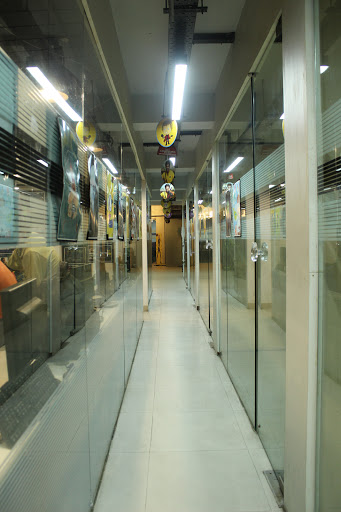The image depicts a long, white-tiled hallway illuminated by bright overhead lights. Lining the hallway are numerous glass doors equipped with see-through handles or doorknobs. Through these glass doors, venetian blinds can be seen, and beyond the blinds, there are benches where people are seated. The hallway extends far into the distance, and there are intersecting passageways that offer additional routes.

The ceiling lights cast a reflective glare on the glass doors, partially obscuring the details of various posters affixed to them. At the end of the hallway, there is a room bathed in warm, orange lighting, providing a stark contrast to the cool, bright ambiance of the corridor. The tiled floor consists of neatly arranged white squares, contributing to the clean and orderly appearance of the space.